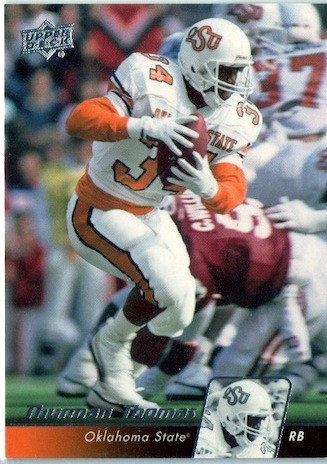The image is an Upper Deck football card featuring Thurman Thomas during his college days at Oklahoma State University. Thomas is depicted in his white Oklahoma State jersey with the number 34, white pants with orange stripes, and a helmet marked with OSU in orange. He is shown carrying the football in both hands, confronting a player in a red jersey, likely from an opposing team, possibly Oklahoma. The upper left corner of the card bears the silver Upper Deck logo, while the bottom displays his name, "Thurman Thomas," in dark blue, followed by "Oklahoma State" and "RB" in white font within an orange to black gradient box. Additionally, there is a small rectangular image of his helmet next to the RB designation, signifying his position as a running back.